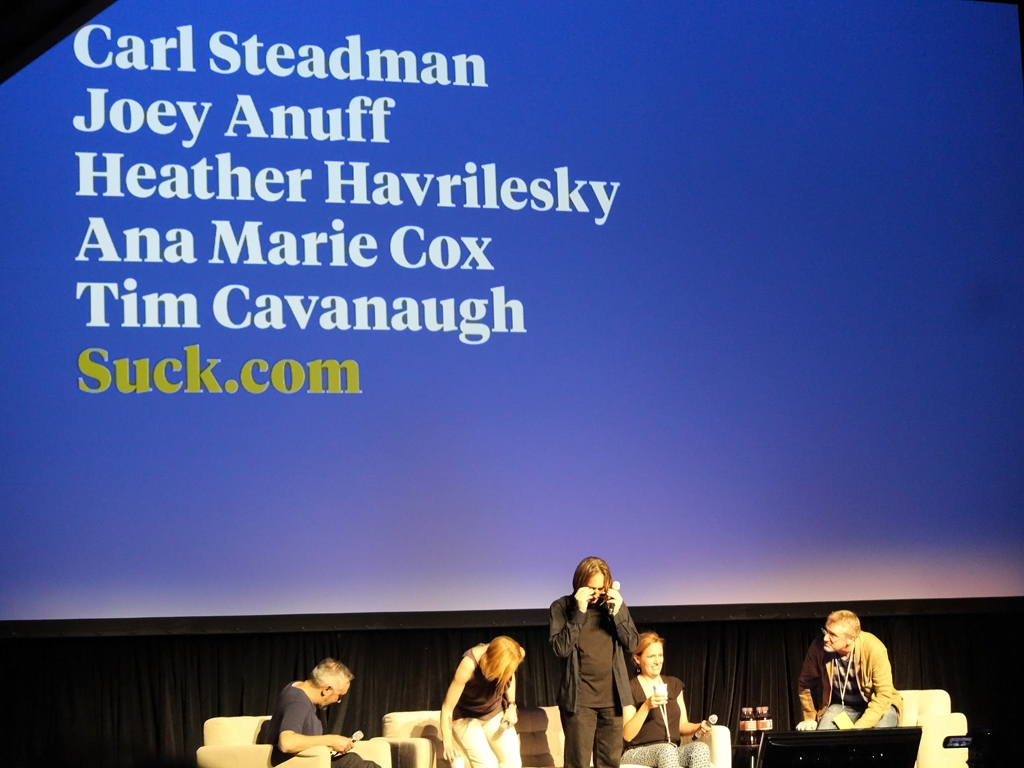This image captures a roundtable discussion or presentation, likely related to or sponsored by Suck.com. Five individuals are either seated or standing on a stage set against a prominent blue background that spans the width of the picture, with a comprehensive banner occupying the upper two-thirds of the frame. The banner in white lettering lists the names Carl Steadman, Joey Anoff, Heather Havrileski, Anna Maria Cox, and Tim Cavanaugh, with 'suck.com' displayed in yellow letters at the bottom.

The lower section of the stage features a black curtain and several white chairs. On the far left, a man in a black T-shirt is seated, holding a microphone. Next to him, a woman in a black shirt and white pants is about to sit down. A person with long hair, wearing a gray sweater, brown shirt, and brown pants is standing, adjusting their glasses with a microphone in their left hand. Behind this individual, a red-haired woman in a brown shirt and white pants also holds a microphone. On the far right, another man in a brown sweater, checked shirt, light-colored pants, and glasses, is about to sit down; he is wearing a lanyard, as is the red-haired woman.

In front of the standing person is a podium, suggesting a formal presentation or discussion setup. The detailed attire and specific actions of each participant indicate a well-coordinated event focusing on or organized by Suck.com.